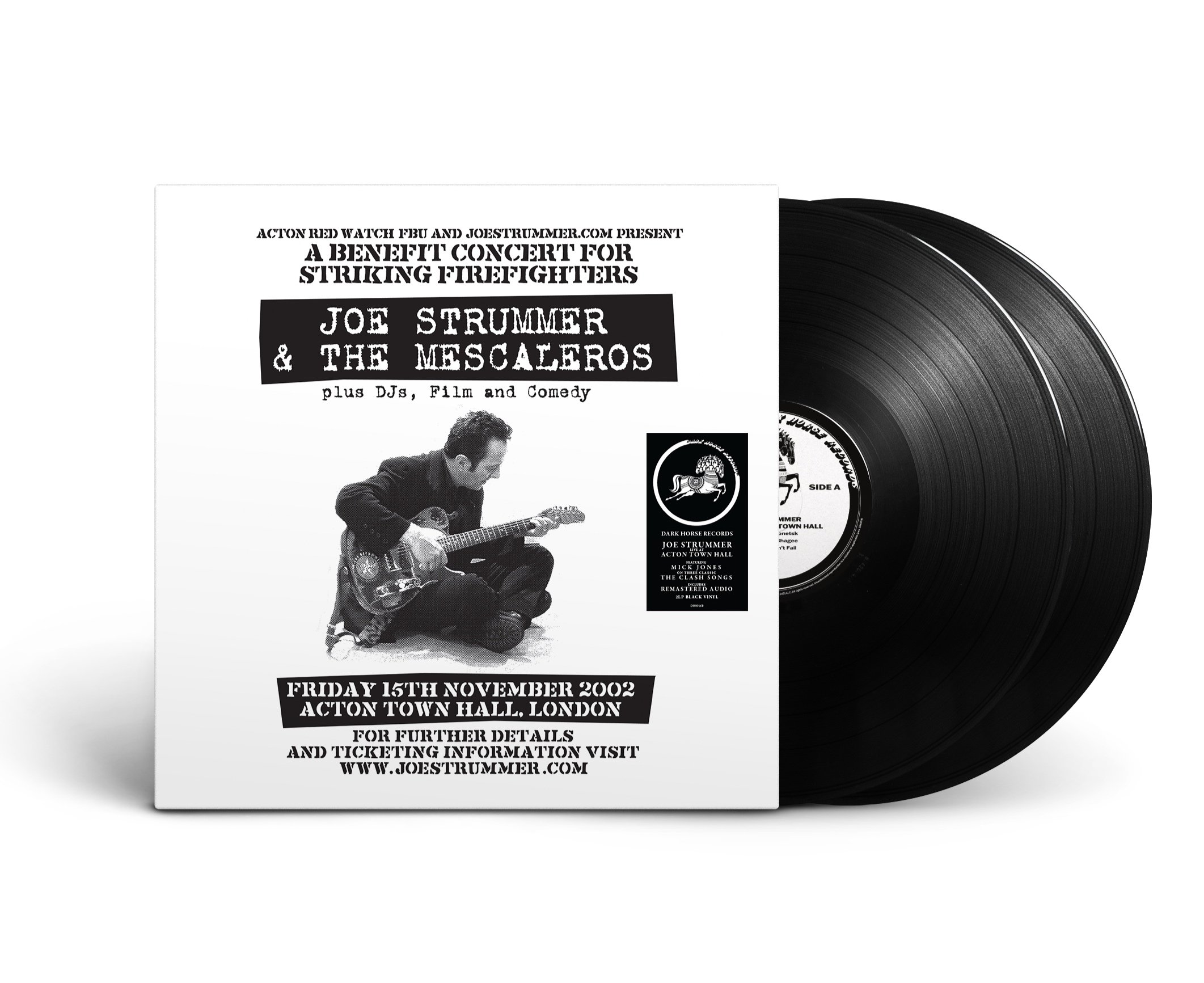The image showcases a black-and-white vinyl album cover, with two half-exposed black records featuring white labels. The album cover, predominantly white, is adorned with black text that reads "Actor Red Watch, Action Red Watch, A Benefit Concert for Striking Firefighters," presented by JoeStrummer.com and the Fire Brigades Union (FBU). Central to the cover is a photograph of a man, possibly Joe Strummer, seated cross-legged in a suit jacket, pants, and black boots, playing an electric guitar. Additional text on the cover highlights "Joe Strummer and the Mescaleros, plus DJs, film, and comedy," along with event details: "Friday, 15th November 2002, Action Town Hall, London." Further information and ticketing details direct viewers to www.joestrummer.com. A small black rectangle on the right side features a white horse image, although the accompanying text is too small to discern.